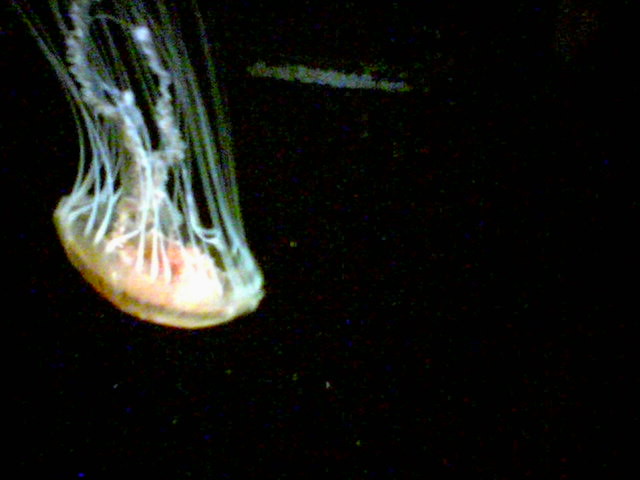The image showcases an East Coast sea nettle jellyfish in the deep oceanic depths. The jellyfish, distinguished by its bright orange-yellow head and predominantly white tentacles, is positioned on the left side of the frame, descending from the upper left corner. Its tendrils and stinging parts flow behind it as it swims downward, almost appearing to be upside down. The background is almost entirely black, creating a stark contrast that emphasizes the jellyfish's vivid colors. A slight row of sea material, possibly floating coral or remnants of a shipwreck, is faintly visible in the distance, adding a subtle layer of mystery to the scene. The image, likely taken by a remotely operated vehicle, hints at movement and depth, further reinforced by the single light source illuminating the descending jellyfish. Overall, the scene exudes a sense of cold, dark isolation, characteristic of the deep ocean environment.